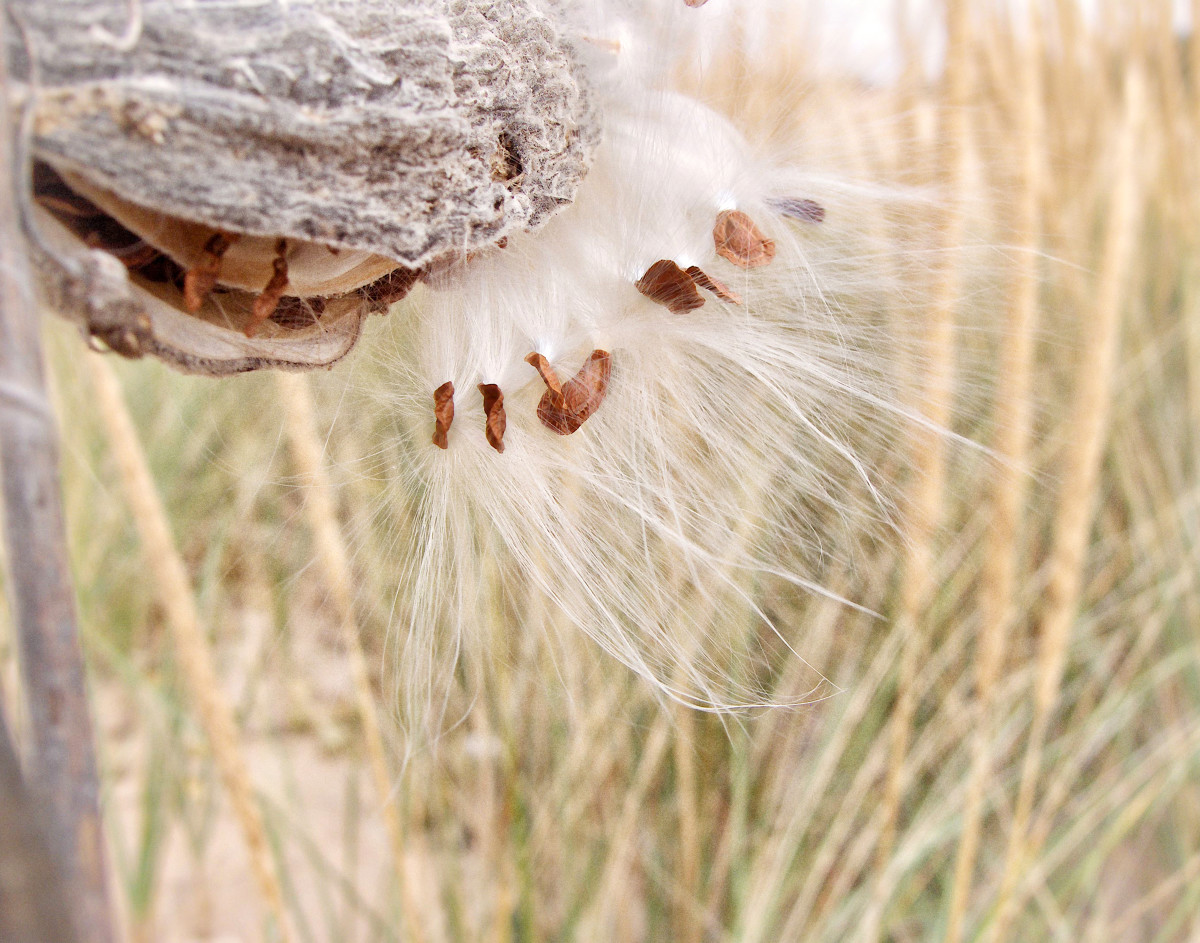The close-up image features a distinctive plant set in an outdoor environment. The plant is primarily brown, varying from medium to darker tones, and transitions from a visible stem on the left to a structure resembling an open clam shell. This opening reveals a lighter brown interior from which long, wispy white strands emerge, akin to fur or the fluff seen on dandelions once they lose their flowers. Within these delicate strands are dispersed brown seed pods, appearing somewhat circular but imperfect. 

The plant seems to be emitting these seeds through the fuzzy material, which is emanating from the brown part of the plant reminiscent of a cracked nut. Surrounding this focal point, the background comprises tall grass that is a blend of green and yellowish-brown, and the ground has a sand-colored hue, hinting at a dry environment. Despite the background grass stalks resembling wheat, they are blurred, emphasizing the sharply focused detail of the wispy strands and the shell-like part of the plant releasing its seeds.